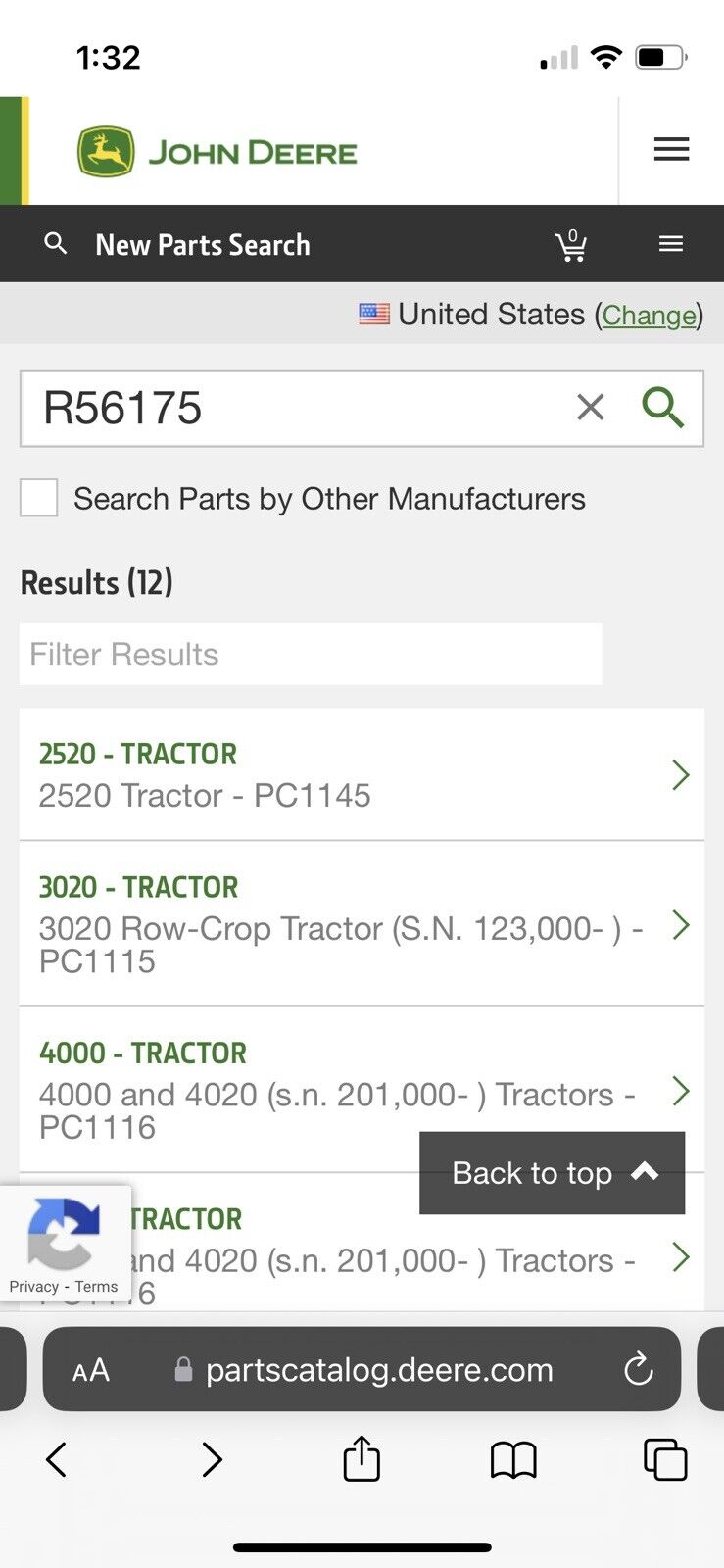This image is a detailed screenshot from a smartphone showcasing the John Deere website. At the top, the white status bar displays essential information: on the left, in black font, the time is shown as 1:32, while on the right, the battery icon indicates a little more than half charge, accompanied by a weak wireless connection symbol, with only one of the four bars lit up, and the Wi-Fi icon.

Below the status bar, the John Deere website header is prominently displayed. "John Deere" is written in bold green capital letters at the top, with the iconic John Deere logo— a yellow deer leaping within a green square with rounded edges—situated to the left of the text. Directly below this is a black navigation menu bar containing the "New Parts Search" option on the left, a shopping cart icon in the center, and a three-horizontal-line icon for a dropdown menu on the right.

The submenu below has a light gray background. It indicates the region as "United States" with a small US flag next to it, followed by the word "Change" in parentheses. Under this, a white rectangle serves as a search box, containing the part number "R56175" in uppercase letters. Just below the search box, it says "Search parts by other manufacturers."

The search results section begins with "Results: 12," displaying the first four of twelve listings. The first result is titled "2520-tractor," followed by entries with more detailed names and numbers. At the very bottom of the page, a gray rectangle with rounded corners contains the website URL, displayed in light gray as "partscatalog.deere.com."